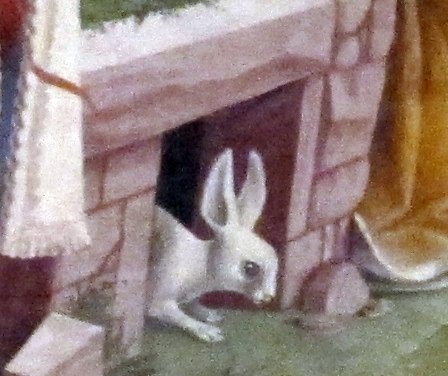This detailed illustration, possibly from a children's book or animated scene, features a diminutive, white rabbit with long, pointy ears and dark brown eyes. The rabbit's slender body and hunched posture hint at a timid or cautious exit through a small, pink stone barrier resembling a fireplace or chimney. The barrier, set between an indoor room with a slate green-gray floor and an outdoor area suggested by green hues at the top, frames the rabbit partially inside with its head, ears, lower legs, and body extending outward. Surrounding the scene, gold and fabric curtains hang on either side, adding a cozy, whimsical touch to the setting.